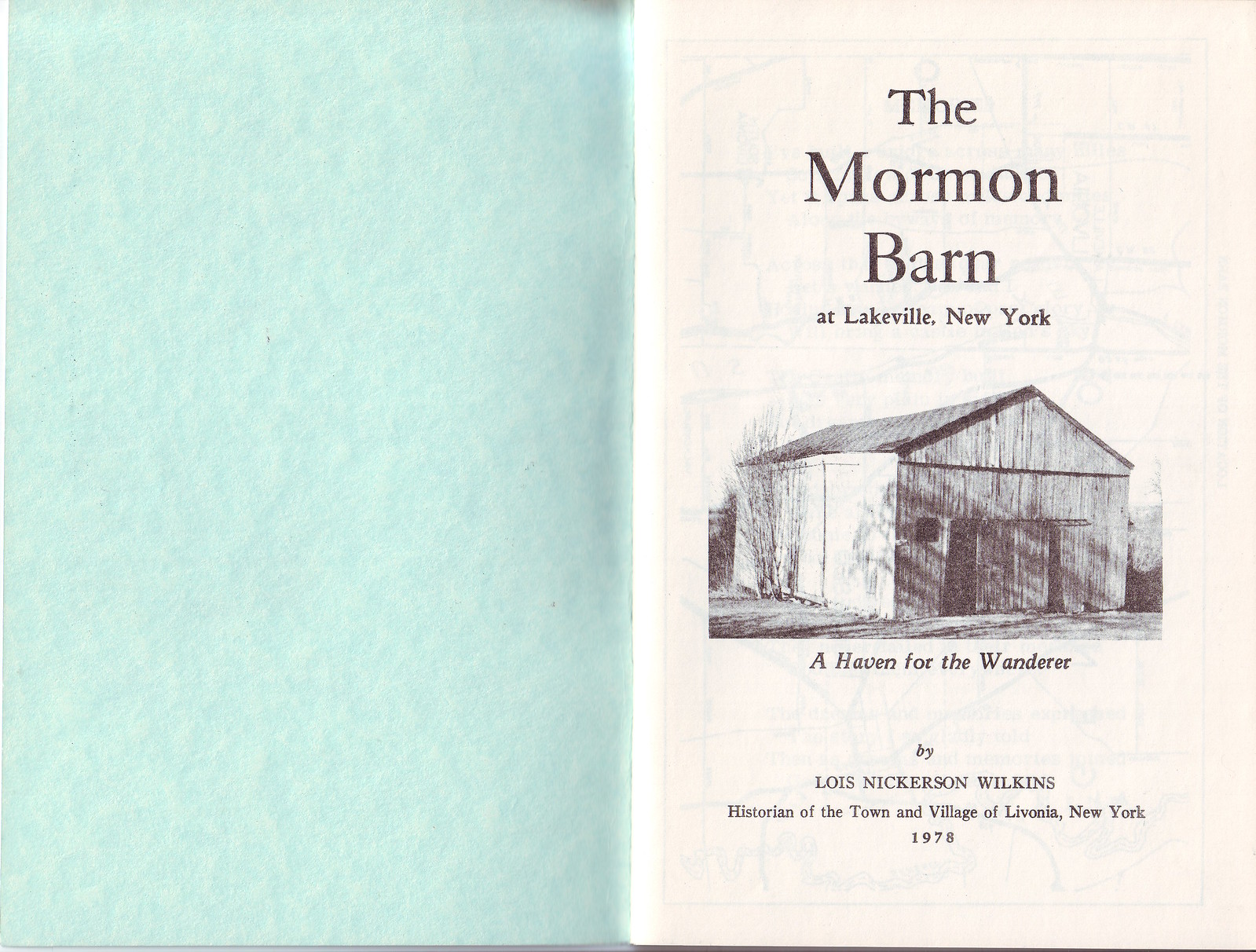The image features an open book displaying its first page alongside the inside of the back cover. The left panel, which is the inside cover, is a light greenish or teal color and is devoid of text. The right panel displays the title page of the book, which has aged to a cream color. Centered on this page is a black-and-white photograph of an old building, likely a barn. Above the photo, the title reads "The Mormon Barn at Lakeview, New York," and below the photo, a caption states "A Haven for the Wanderer." At the bottom of the page, there is a citation which reads, "By Louis Nickerson Wilkins, Historian of the Town and Village of Livonia, New York, 1978."